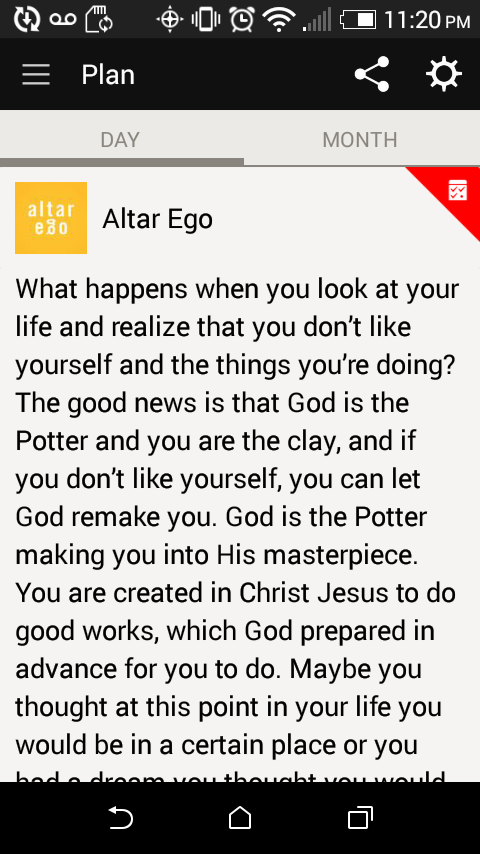The image is a detailed screenshot of a cell phone display featuring an open app named "Alter Ego." The time on the phone reads 11:20 p.m., and the battery icon indicates it's at about 50% charge. The app has a white background with black text, and at the top, a yellow logo with the words "Alter Ego" in white is prominently displayed. The main text in the app revolves around self-reflection and spiritual guidance, stating: "What happens when you look at your life and realize you don't like yourself and the things you're doing? The good news is that God is the potter and you are the clay. If you don't like yourself, you can let God remake you. God is the potter making you into his masterpiece. You are created in Christ Jesus to do good works which God prepared in advance for you to do." It suggests that despite current disappointments or unmet dreams, there is hope for transformation through divine intervention. At the bottom of the screen, typical navigation icons are visible, including an undo/back arrow, a home button, and a multitasking button with two overlapping squares. The overall design and content of the app focus on spiritual self-improvement and resilience.